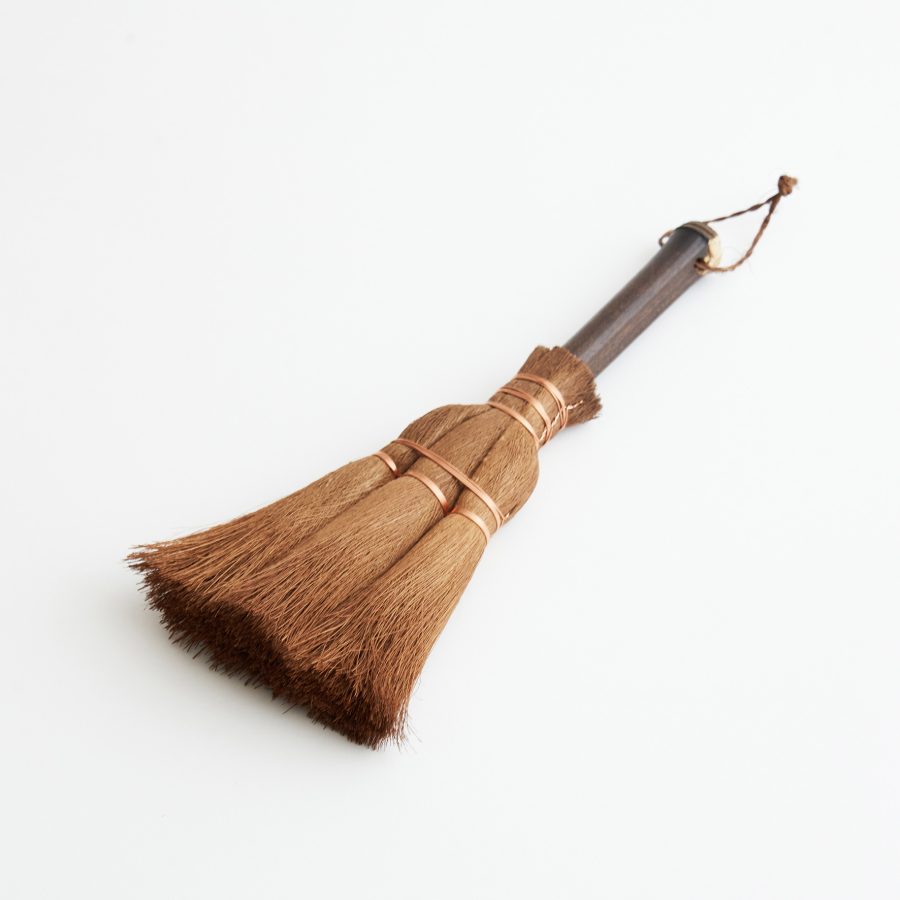This photograph features a meticulously detailed antique-style broom, lying against a plain white background, devoid of any shadows or additional colors. The broom, appearing very small and almost toy-like in scale, has a rich brown, extremely short handle, approximately the same length as the broom head itself. This handle, crafted from dark textured wood, is capped with what appears to be golden or possibly ivory material, and features a small brown string looped through a hole at the top, suggesting it was designed to be hung. 

The broom head is attached to the handle and is composed of thick, coarse, light brown straw bristles. These bristles are secured in place by multiple bindings of copper wire or golden ribbons, located at the base and further down the length of the bristles. This bundling method contributes to a thick, shaggy appearance and ensures the structural integrity of the broom. The overall design and craftsmanship hint at an aged, antique aesthetic, possibly indicating that this broom may serve more as a decorative piece or a model rather than a functional cleaning tool.